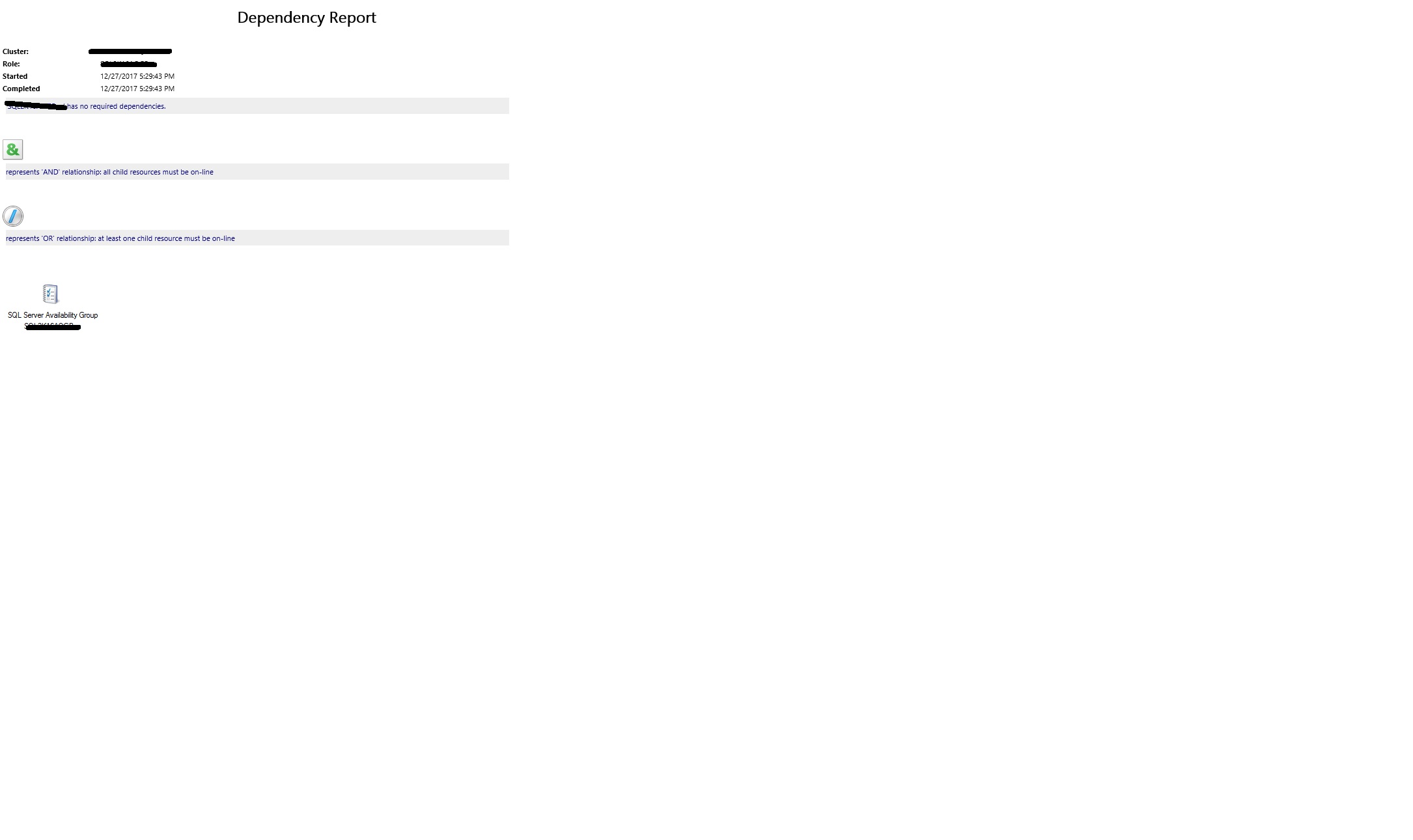The image displays a "Dependency Report" screen from a computer. At the top and in black font, the heading "Dependency Report" is clearly visible in the upper left corner. Below this heading, there are labeled sections for "roles" and another word that is too small to decipher. Both these sections have been crossed out, and the data to the right of them has also been obscured. 

Further down, there are timestamps indicating when the process was "Started" and "Completed," both showing December 27th, 2017 at 5:29 PM, suggesting the task started and finished instantaneously. Below these timestamps, there is a partially redacted sentence which ends with the phrase "has no required dependencies."

Following the sentences, there is a graphical legend with symbols. One symbolic box, marked with an ampersand (&), explains that it "represents AND relationship; all child resources must be online." Another symbol, a circle with a blue line, illustrates an "OR relationship; at least one child resource must be online."

At the bottom of the image, there is an icon resembling a folder with the label "Server Availability," indicating this section provides information on the operational status of various servers.

This detailed caption provides a comprehensive overview of the various elements and information presented in the image.